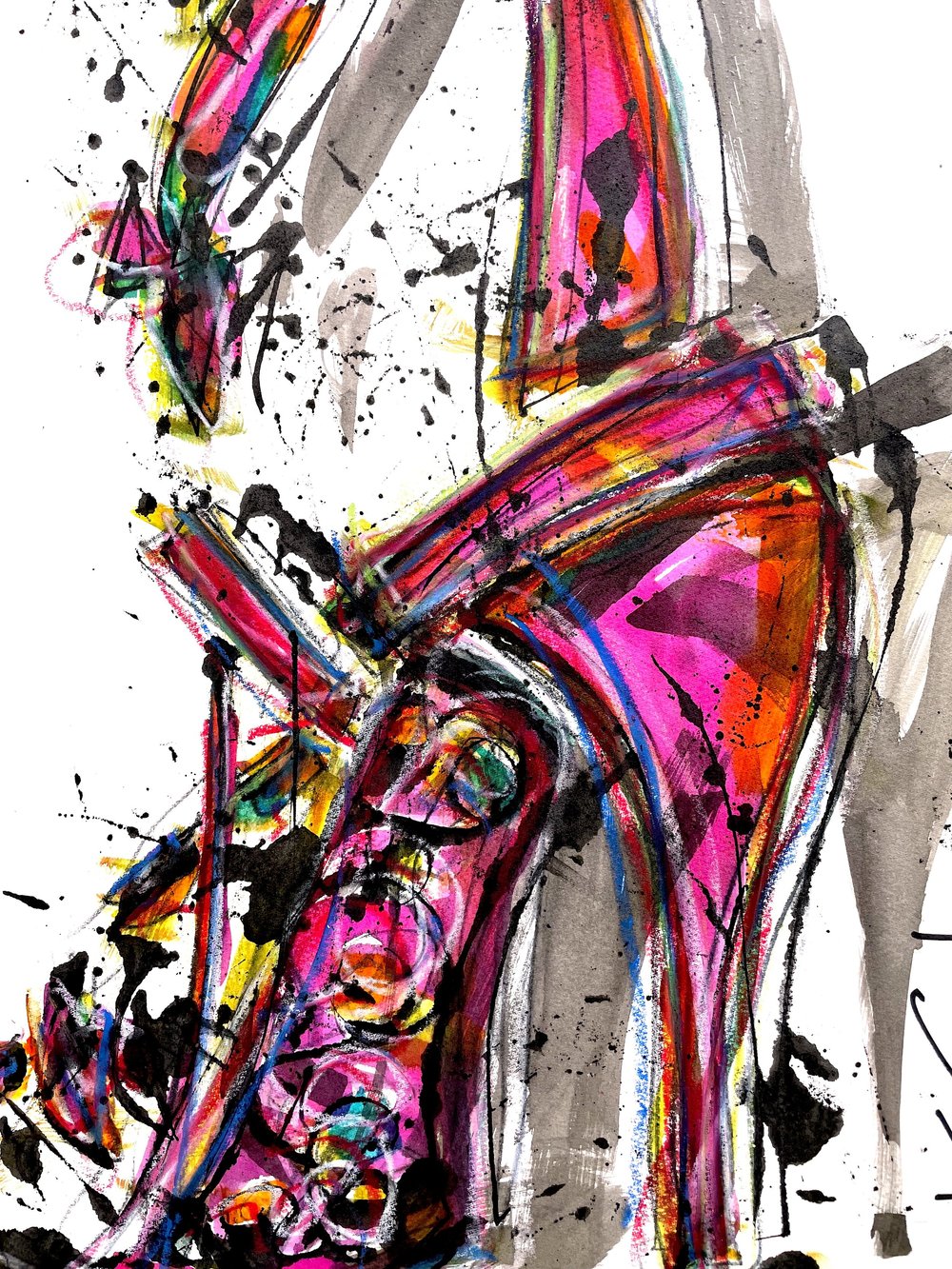The painting is a vertically oriented abstract artwork with a primarily white background. Central to the canvas is a collection of splotches and streaks, predominantly in hot pink, but also featuring red, blue, black, white, yellow, green, and orange. An upside-down triangular shape stands out in the middle, created with chalky textures and watercolor-like mediums. Above this triangle, a horizontal line extends halfway across the canvas before merging into another triangular form composed of chaotic streaks, adding to the piece's abstract nature. On the bottom left, there’s a prominent blue trunk-like shape with white spirals, enhancing the texture and detail in that area. Thin, thick, and rectangular gray strokes are visible predominantly on the right side, contributing to the painting's industrial feel. The inclusion of purples, black splatters, and random elongated lines suggest the artist's freeform and unstructured approach. The top left corner features additional detailed spirals and shapes, layering complexity into the background dominated by a few gray streaks.